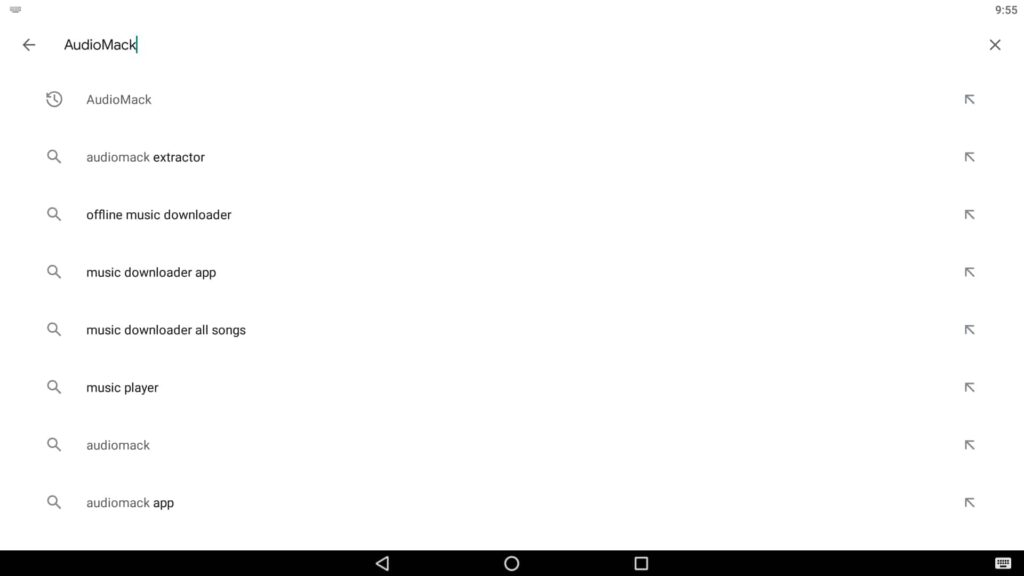The image displays a user interface with a predominantly white background, approximately 50% wider than it is tall. In the upper right corner, the time "9:55" is displayed, with an "X" icon below it. On the left-hand side, there is a grey left-pointing arrow icon next to the text "Audiomack" in black, followed by a blinking cursor, indicating an active search bar.

Below this search bar, the content is indented. The first line features a time icon alongside the text "Audiomack." Each subsequent line is paired with a gray arrow pointing toward the upper left. The following lines include:
- A magnifying glass icon next to the text "Audiomack Extractor"
- A magnifying glass icon next to the text "Offline Music Downloader"
- A magnifying glass icon next to the text "Music Downloader App"
- A magnifying glass icon next to the text "Music Downloader All Songs"
- A magnifying glass icon next to the text "Music Player"
- A magnifying glass icon next to the text "Audiomack"
- A magnifying glass icon next to the text "Audiomack App"

This suggests a search functionality for various Audiomack-related queries. At the bottom of the image, there is a horizontal black bar encompassing roughly 5% to 7% of the image's height. Centered within this bar are three icons: a left-pointing triangle, a circle, and a square, likely representing media controls.

Overall, the image appears to depict a search interface for an Audiomack-related application or website, with various music downloading and playing options listed.